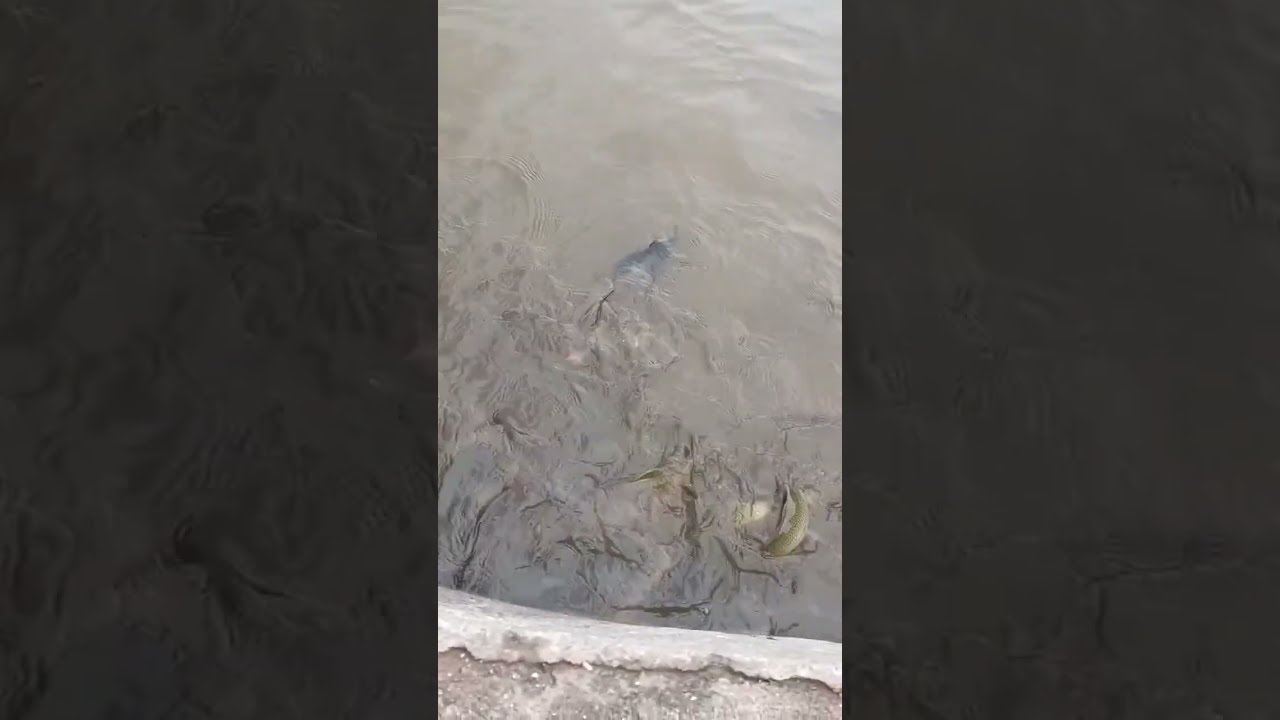The image captures a bird's-eye view of a murky, opaque body of water, with a grayish-white stone or concrete ledge visible at the bottom edge of the frame, suggesting the photograph was taken from a platform or shore. The water appears brown and muddy, slightly disturbed with ripples indicating a windy environment. Just north of the center of the image, a dark-colored object, possibly a larger fish, is partially submerged and visible through the murky water. Additionally, a beige-colored object is seen towards the bottom right, though its details are unclear. Along the shoreline, several fish with greenish hues are clustered together, some partially emerging from the water. The overall scene is devoid of boats or people, and the primary colors consist of dirty tan water and the white and gray tones of the stone.